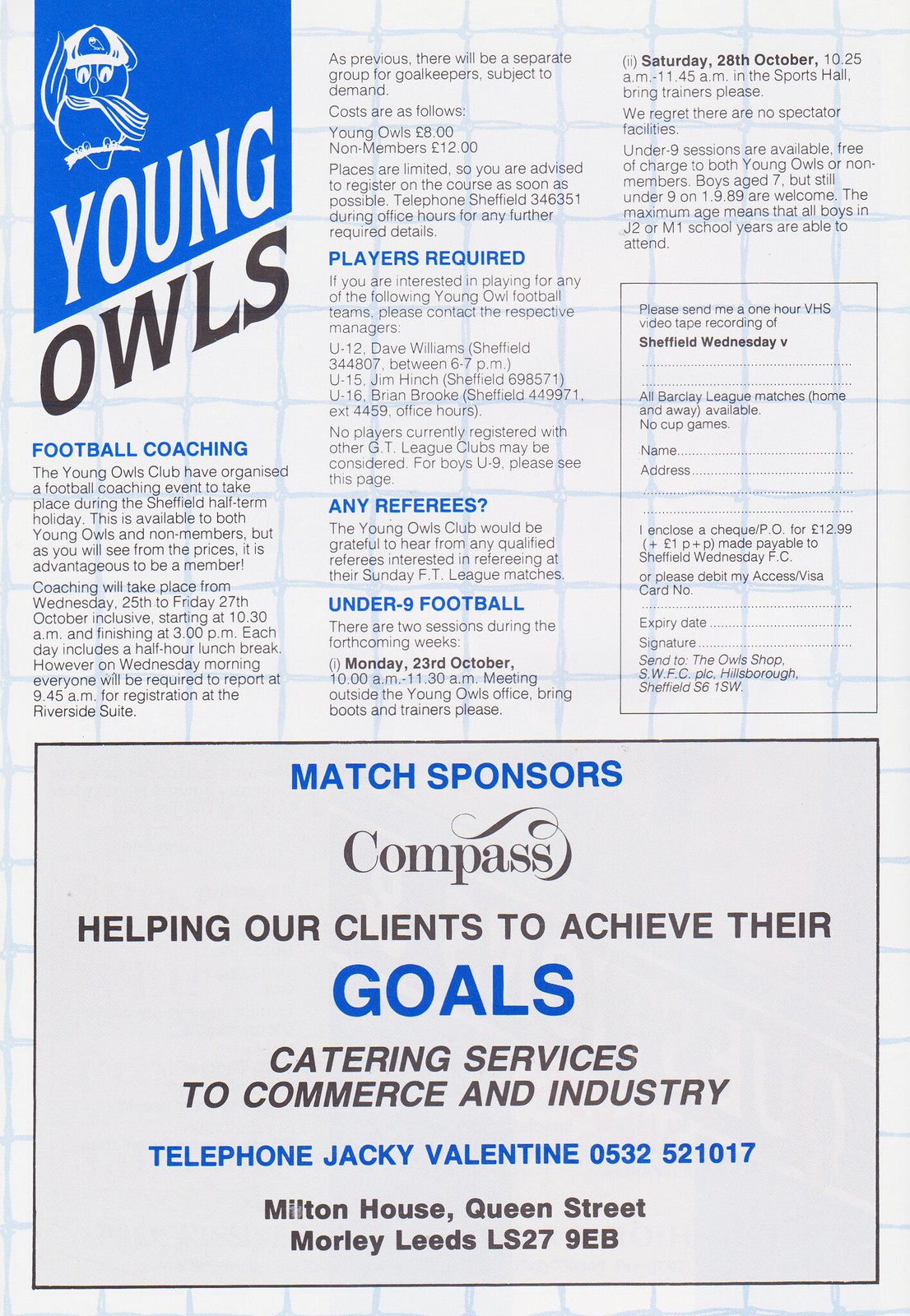The poster for the Young Owls Football Club prominently features a vibrant header in the upper left corner, reading "Young Owls" with the word "Young" in white font against a blue background and "Owls" in black font. A cartoon owl, clad in a cap and scarf, perched on a branch, sits beside the text, giving a playful and inviting appearance. Below this, the poster details several highlighted sections, each with informative text.

Firstly, the "Football Coaching" section outlines a coaching event set for the Sheffield half-term holiday. It welcomes both members and non-members, though members benefit from reduced registration fees (£8 for members, £12 for non-members). Taking place from Wednesday, October 25th to Friday, October 27th, the event runs from 10:30 a.m. to 3 p.m. each day, with a half-hour lunch break. Notably, participants are required to report at 9:45 a.m. on Wednesday for registration at the Riverside Suite, with a dedicated group for goalkeepers pending demand. Interested individuals should register promptly as spots are limited, by calling Sheffield 346351 during office hours.

The "Players Required" section invites boys interested in joining specific Young Owl football teams to contact respective team managers. The teams and corresponding contacts are: U12 - Dave Williams (Sheffield 344807, 6-7 p.m.); U15 - Jim Hench (Sheffield 698571); and U16 - Brian Brooke (Sheffield 449971, ext. 4459, office hours). Boys under 9 must register by January 9th, 1989, ensuring they fall within the age group of J2 or M1 school years.

The "Any Referees" section seeks qualified referees for Sunday FT League matches, while the "Under 9 Football" section provides details for two forthcoming training sessions for boys aged 7 to under 9, free for both members and non-members. Sessions are on Monday, October 23rd from 10 a.m. to 11 a.m. (meeting outside the Young Owls office) and on Saturday, October 28th from 10:25 a.m. to 11:45 a.m. (in the sports hall).

Towards the bottom of the poster, enclosed in a bordered section with a light gray background, are details of the match sponsors. Headlined by "Match Sponsors" in blue font, it highlights "Compass" with the motto "Helping Our Clients to Achieve Their Goals" and "Catering Services to Commerce and Industry." Contact information for Jackie Valentine (05-32-52-10-17) and an address (Milton House, Queen Street, Morley Leeds, LS279EB) are provided beneath.

The overall design integrates a clean white background complemented by blue squares that evoke a fencing pattern, enhancing the visual appeal of the information-rich poster.